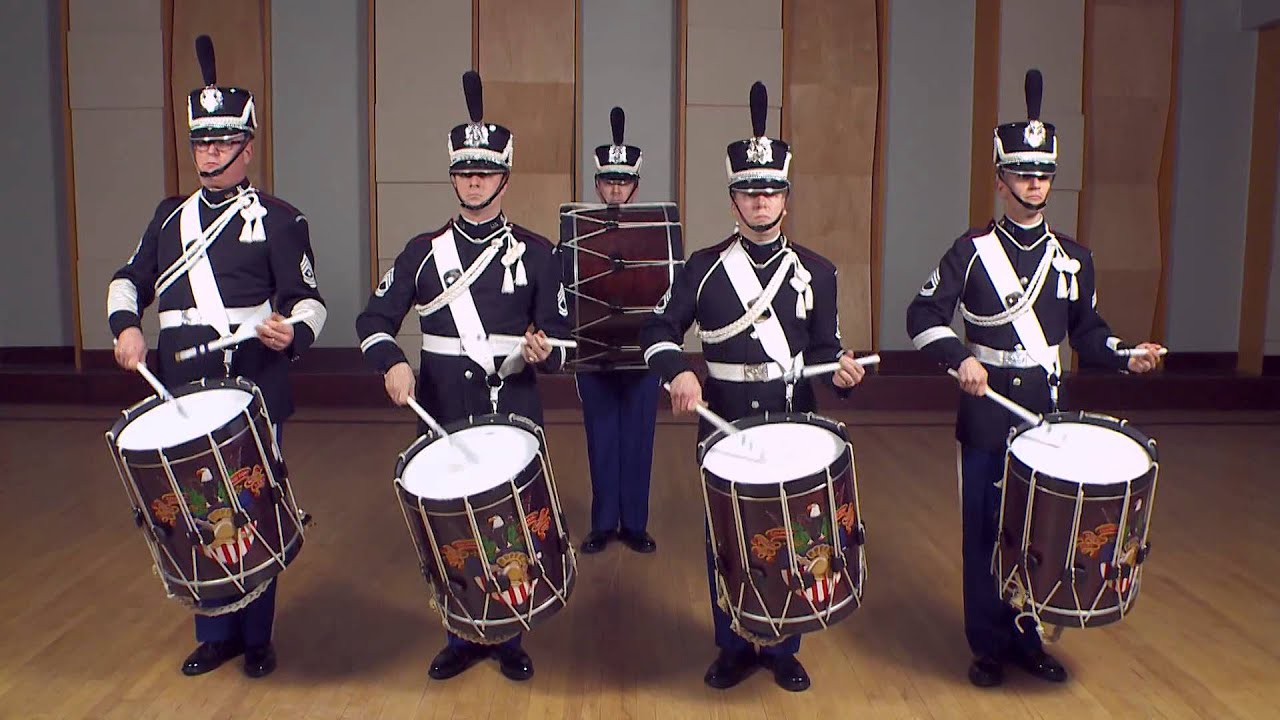In this color photograph, a military drum corps is depicted in detailed formation within a musical studio environment. The image features five male soldiers dressed in antiquated military uniforms that consist of black upper garments, black pants, and black shoes. Their uniforms are accented with white sashes across their chests, white cuffs on their sleeves, and intricate black helmets adorned with white embroidery and large black crests. Four soldiers in the front row are playing large snare drums with white drumheads and an insignia that resembles a bald eagle with an American flag, while a fifth soldier stands in the background, partly obscured by a mahogany-colored bass drum strapped to his chest. The stoic expressions on their faces and their erect posture contribute to their formal and disciplined appearance.

The background suggests the setting is inside a musical studio or recreation building, featuring light blue or off-gray walls with sound-deadening pads in various shades of blue, pink, and orange. The floor appears to be wooden or laminate with a distinctive wood grain. Eight visible rows of sound-dampening material line the walls, enhancing the acoustics for the musicians. The soldiers appear to be sergeants, as indicated by arm patches on their uniforms. The scene captures the precise and ceremonial nature of the military drum corps, with each member in perfect alignment and rhythm.